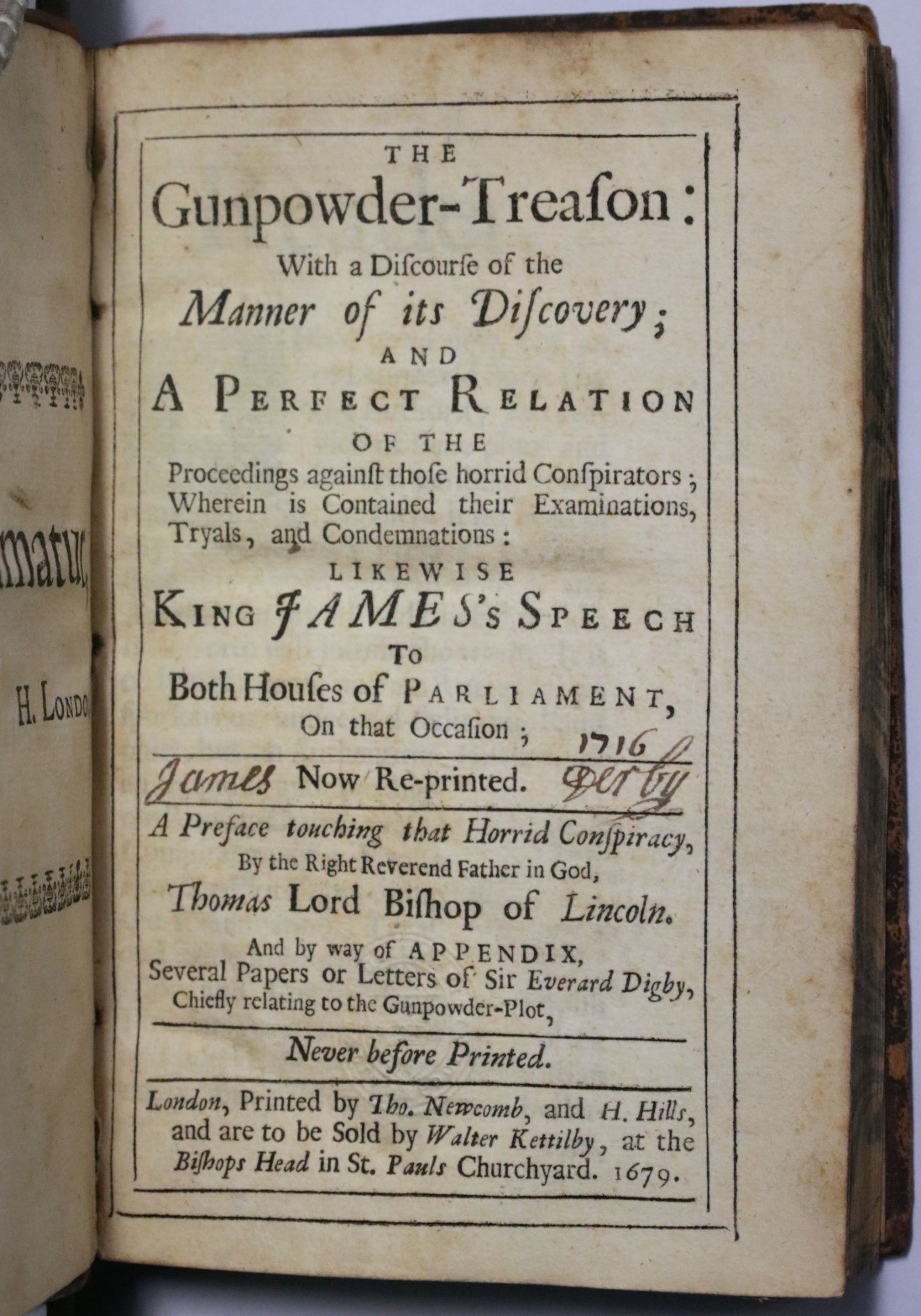The image depicts a very old, open book with an aged, hard leather cover. The right page, fully visible, is stained with age and covered in writing from an old English style. The prominent text reads, "The Gunpowder Treason, with a Discourse of the Manner of its Discovery, and a Perfect Relation of the Proceedings Against Those Horrid Conspirators. Wherein is contained their examinations, trials, and condemnations. Likewise, King James's speech to both Houses of Parliament on that occasion. Now reprinted." In the center, it indicates "1716 Derby," followed by "Never before printed." Additional text at the bottom attributes the work: "Printed by Doe, Newcomb, and H. Hills, and sold by Walter Kettleby at the Bishop's Head in St. Paul's Churchyard, 1679." To the left, there is mention of the right reverend father in God, Thomas Lord Bishop of Lincoln, and an appendix including letters of Sir Everard Digby relating to the Gunpowder Plot.